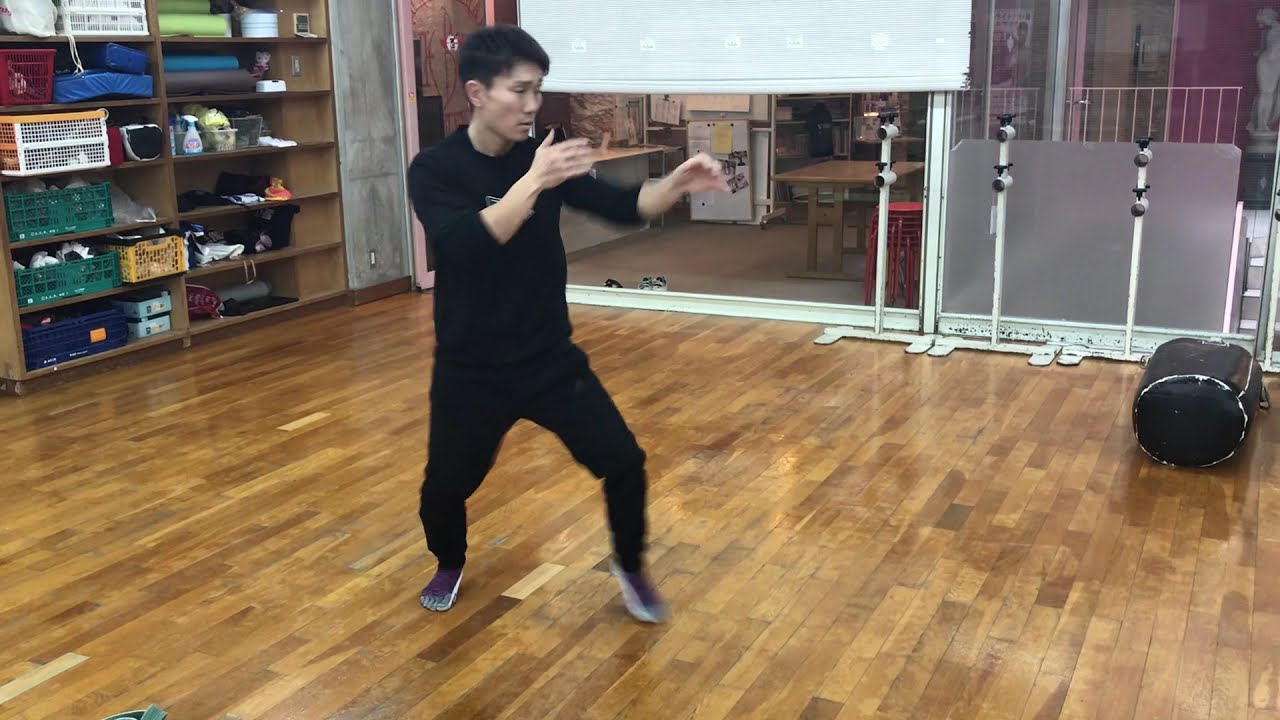This photograph captures a young, clean-shaven Asian man with short dark hair practicing martial arts in a spacious indoor training center. He is wearing a black pull-sleeve t-shirt and black trousers paired with distinctive purple and white socks. Positioned in a fighting stance, he has his hands raised in front of him and is balanced on his tiptoes, with his weight shifted onto his back leg. The room features a wooden plank floor and is illuminated by floor-to-ceiling glass windows with partially drawn curtains. Behind him, there are shelves filled with various training equipment, including mats, storage bins, and a spray bottle. Additionally, there are cylindrical black objects and metal stands near the glass windows that appear to be part of the training apparatus.